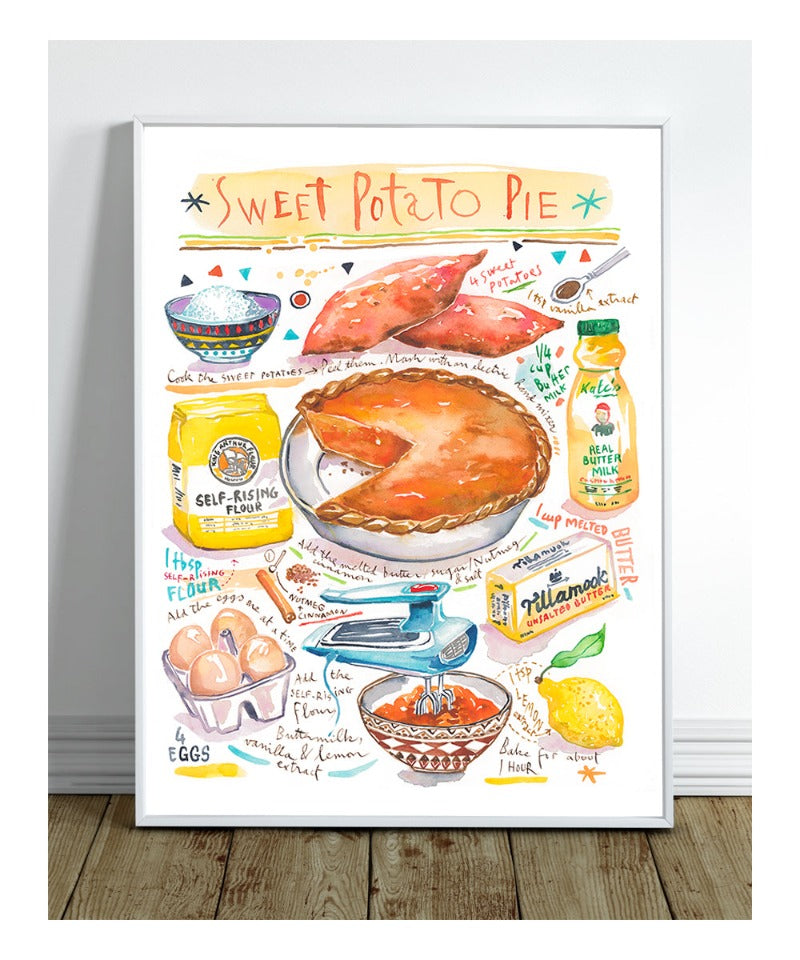This framed artwork sits against a white wall on a wooden floor and features a white frame with a white background. The detailed and colorful illustration portrays the ingredients and steps to make sweet potato pie, presented almost like a recipe. The title "Sweet Potato Pie" is written in cursive at the top in brown letters with a beige stripe underneath. At the center of the artwork is a brownish sweet potato pie with a slice cut out. Above it are two stacked sweet potatoes. 

The upper left corner shows a bowl of flour, while the upper right displays a spoon filled with either cinnamon or nutmeg. Below, a bottle of real buttermilk and a self-rising flour packet in yellow and white are depicted to the left of the pie. In the lower left corner, an egg carton with four eggs is detailed, and the lower right corner shows a whole lemon with a leaf and a stick of butter. There is also a mixing bowl with brown batter being blended by a blue mixer. Scattered across the canvas are additional ingredients like a bag of flour, an egg beater, and instructions written in cursive, making the text hard to read but adding a personal touch. This richly detailed painting captures all the components needed to create a sweet potato pie, visually narrating the recipe with a blend of artistry and practicality.